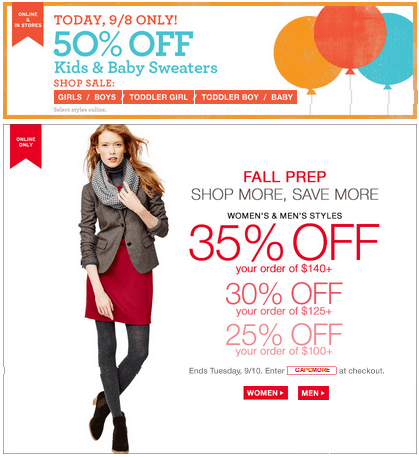This advertisement screenshot showcases a detailed sale event featuring multiple offers across various clothing categories. The top portion of the graphic prominently displays three colorful balloons—orange, red-orange, and teal—on the right side. The central message announces a special sale, offering a 50% discount on kids' and baby sweaters both online and in-store, limited to today only, with availability for girls, boys, toddler girls, and toddler boys/babies. 

The bottom section of the advertisement highlights a 'Fall Prep' promotion involving discounts on women's and men's styles. The offer details are outlined as follows:
- 35% off orders of $140 or more
- 30% off orders of $120 or more
- 25% off orders of $100 or more

An image of a woman wearing a red dress, a scarf, and black pants or leggings accompanies the text. Further instructions mention that this offer ends on Tuesday, and there's a reminder to enter a promotional code at checkout for the discount, though the specific code appears to be blurred out. A prominent red button likely serves as a link to women's and men's categories.